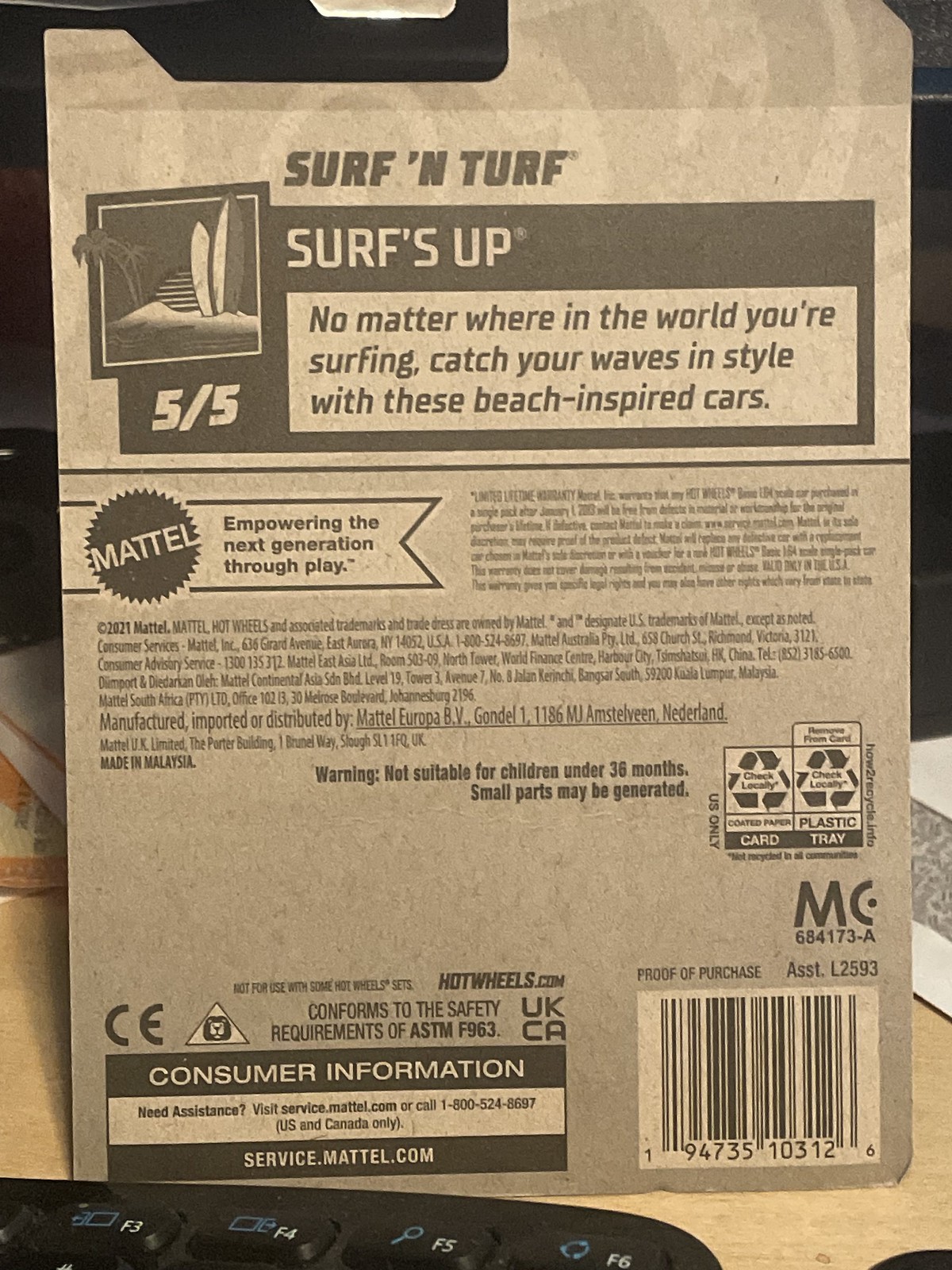This image is a close-up of the back of a Mattel toy product page, presented in a grayed-out or brown cardboard material. At the very top, the text reads "Surf and Turf." Below this, there is a black or dark gray rectangle with the white text "Surf's Up." To the left within this black rectangle, there is an illustration of a small stamp featuring a beach scene with two surfboards on the right and two palm trees on the left. Further to the left, it says "5/5" and there is a ribbon-like graphic with "Mattel" in white text, followed by the phrase "Empowering the next generation through play."

On the right side of the black rectangle, a white rectangle holds the text: "No matter where in the world you're surfing, catch your waves in style with these beach-inspired cars." Below this line, there is a Mattel emblem followed by various small text and symbols. Among the legible text, it includes a safety warning: "Warning, not suitable for children under 36 months. Small parts may be generated," and consumer information: "Need assistance? Visit service.mattel.com or call 1-800-524-8697 (US and Canada only)." There are also recycling icons and, in the bottom right corner, a barcode, while the bottom left corner has a rectangle labeled "Consumer Information" with additional support details.